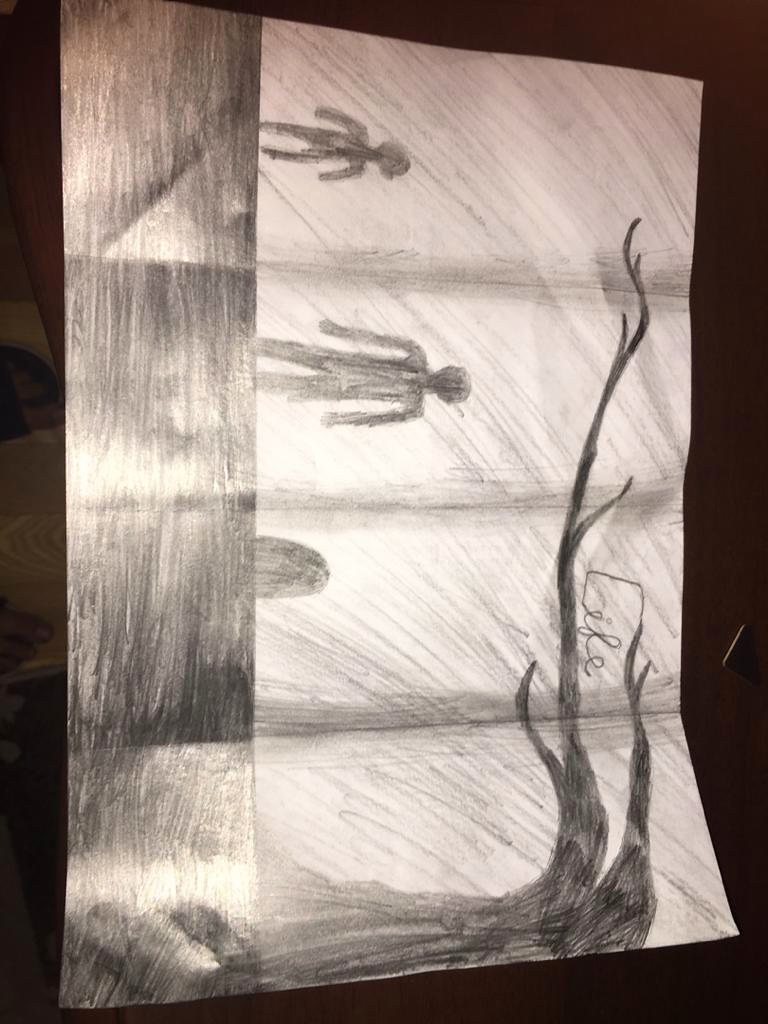This vertical sheet of white paper, folded into four equal rectangular parts in a brochure format, contains a detailed black and white pencil drawing. The artwork, although tilted to the right, prominently features the word "life" written sideways in cursive, extending above dark, leafless tree branches that bend to the right side of the image.

On the left side of the image, vertical lines create the appearance of a textured ground or base, the exact origin of which is ambiguous. Situated on this ground are rudimentary stick figures, depicted in the first and second columns. These stick figures have no distinct gender characteristics. Above them, light gray streaks suggest an overcast sky.

The stick figures appear to be positioned before a black, half-oval shape resembling a gravestone. The first stick figure is shorter in stature, while the second is slightly taller. This sequence, starting with the two figures and culminating in the gravestone, seems to symbolize the passage of life stages—from childhood (the shorter figure) to adulthood (the taller figure), and finally, to death (the gravestone).